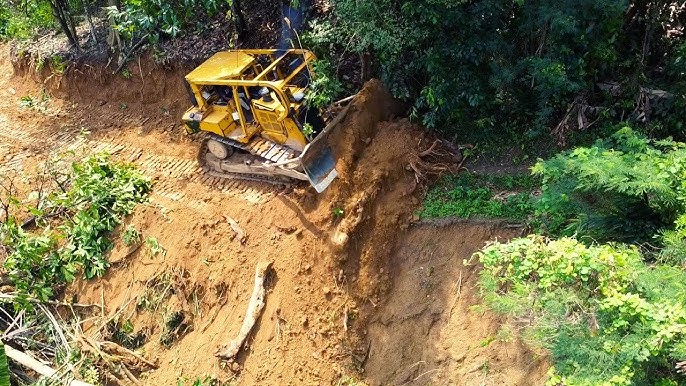The photograph captures a yellow bulldozer, equipped with a large scoop on the front, pushing brown, clay-like dirt along a steep dirt embankment, likely in an effort to build or repair a road. It appears to be an outside shot, perhaps from an aerial viewpoint, displaying the machine in motion. The scene is quite dramatic, with the bulldozer precariously positioned on what seems to be a very steep slope, creating a tense, uneasy feeling as if it might tip over. Numerous green trees, weeds, and forest underbrush including logs, branches, sticks, and leaves surround the area. The tracks already cleared by the bulldozer are visible to the left, indicating significant progress in the dirt-moving task. The driver remains unseen and the dirt being moved flows from left to right across the image.